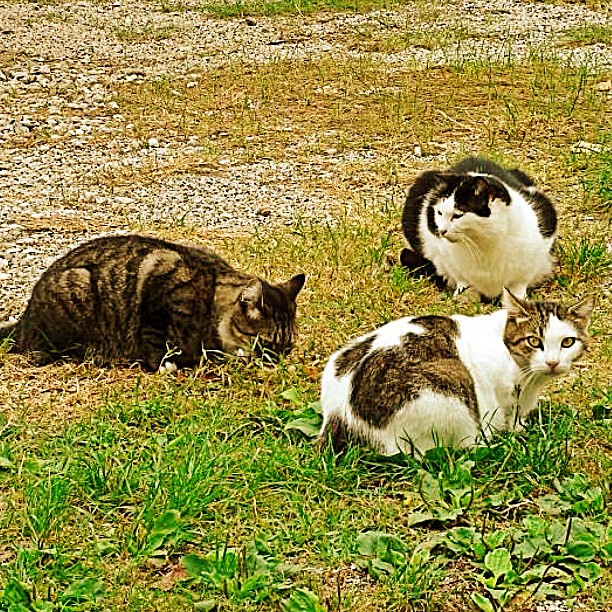This outdoor photograph captures a tranquil scene of three cats lounging on a patchy, grassy field. The foreground features a distinctive cat with white fur and large brown patches, including a half-brown, half-white face with alert, brown eyes directed at the camera. Directly behind, slightly to the right, is another cat predominantly white with black spots. This cat, sitting upright, faces forward but has its head slightly turned to the left, possibly observing the scene or the other cats. The third cat, situated to the left and slightly behind the first, presents a contrast with its brown fur adorned with dark stripes. It lies with its head down on the ground, possibly napping. The grass ranges from green to dry yellow patches, lending a rustic feel to the setting. Despite the image's low resolution, the distinct colors and positions of the cats create a compelling and endearing snapshot of these feline companions.